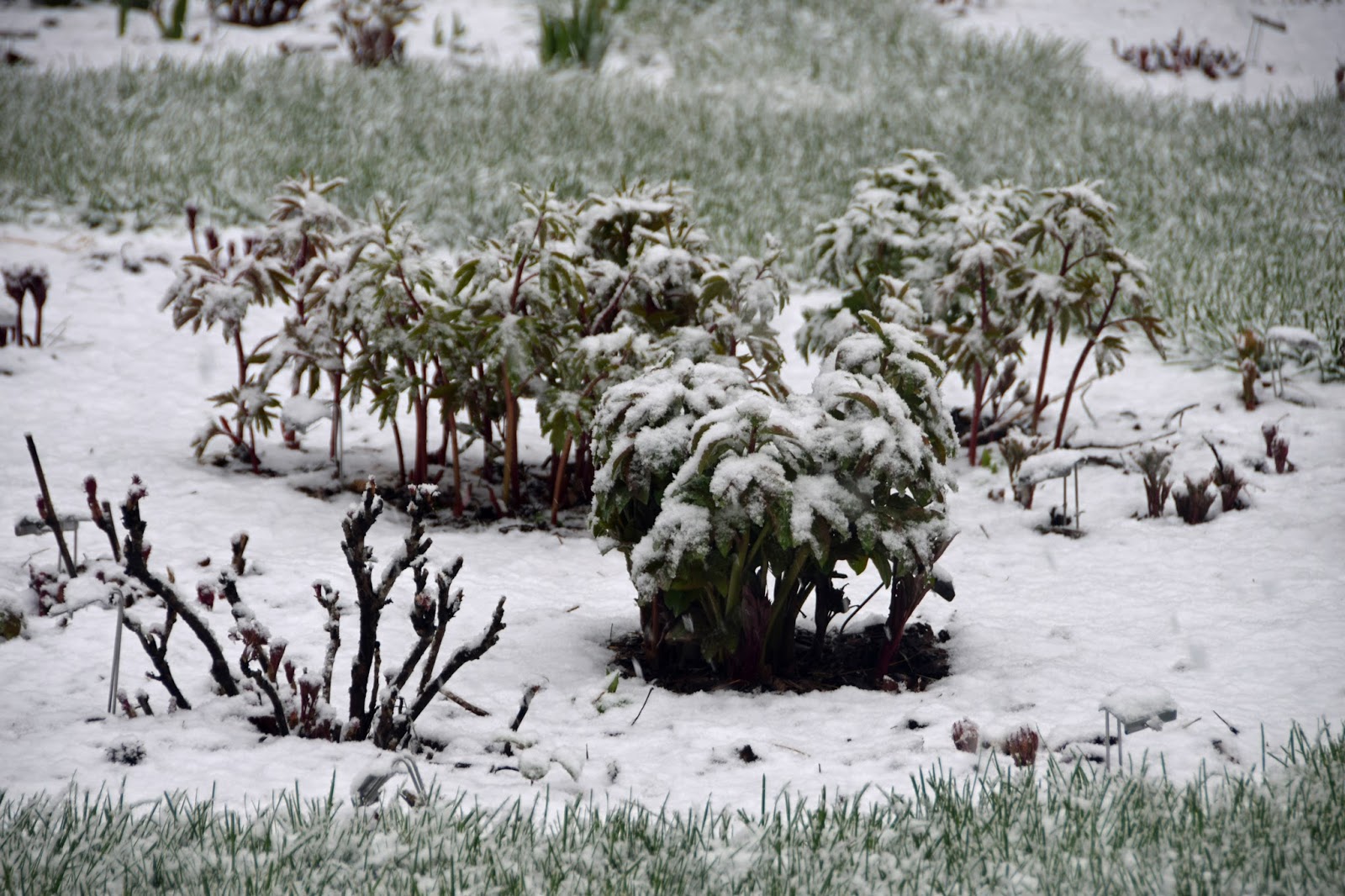This horizontal, rectangular photo captures a winter landscape bathed in daylight, with a muted, grayish tone that suggests a rather dim day. The foreground features an icy, partially snow-covered field of longer grass, interspersed with snow patches of varying depths. Dominating the middle of the scene are small bushes, laden with snow that weighs down their green, leaf-covered branches. Sporadic brown sticks and black branches poke up through the white, adding textural contrast. Further back, behind the bushes, lies another stretch of grass and a slope enveloped in more snow. The snow appears to be denser in some areas than others, particularly toward the top right and left corners of the photo. Small pine cones are scattered at the bottom of the image, adding additional detail to the wintry tableau.